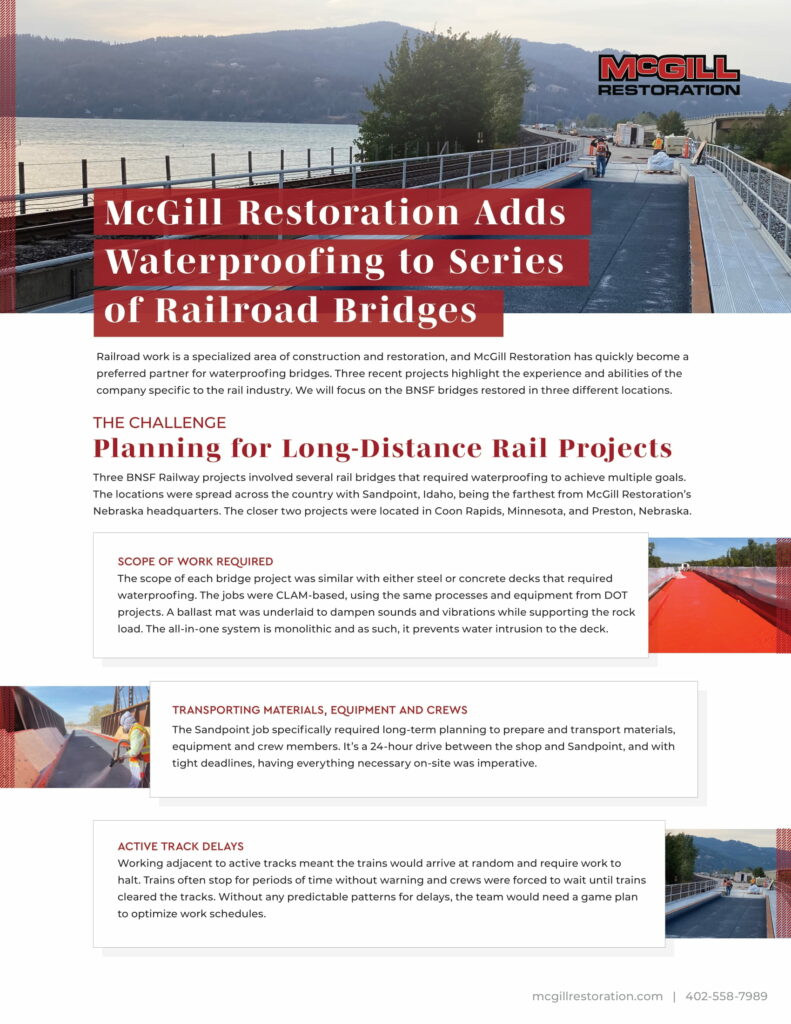This image is a detailed advertisement or brochure by McGill Restoration, focusing on their specialized work in waterproofing railroad bridges. The top third of the rectangular layout prominently features a picturesque scene: a bridge under construction over a body of water, with a distant mountain range, lush trees, and white railings on either side. Visible on the bridge are workers in yellow safety vests and a white car with its back door open. The top right corner of the image displays the McGill Restoration logo.

The main title, "McGill Restoration adds waterproofing to a series of railroad bridges," is boldly written in white text with a red background. Below that, the text elaborates on the specialized nature of railroad work and highlights McGill Restoration's reputation and recent projects, including three BNSF bridges. There are specific sections detailing "The challenge planning for long distance rail projects," "Scope of work required," "Transporting materials, equipment, and crews," and "Active track delays," each accompanied by relevant images. Smaller pictures pepper the layout, including a red bridge to the right and construction scenes to the left and bottom. The bottom of the advertisement provides contact details, including the website MacGillRestoration.com and phone number 402-558-7989. Overall, the image serves as a comprehensive showcase of McGill Restoration's work and expertise in the field.